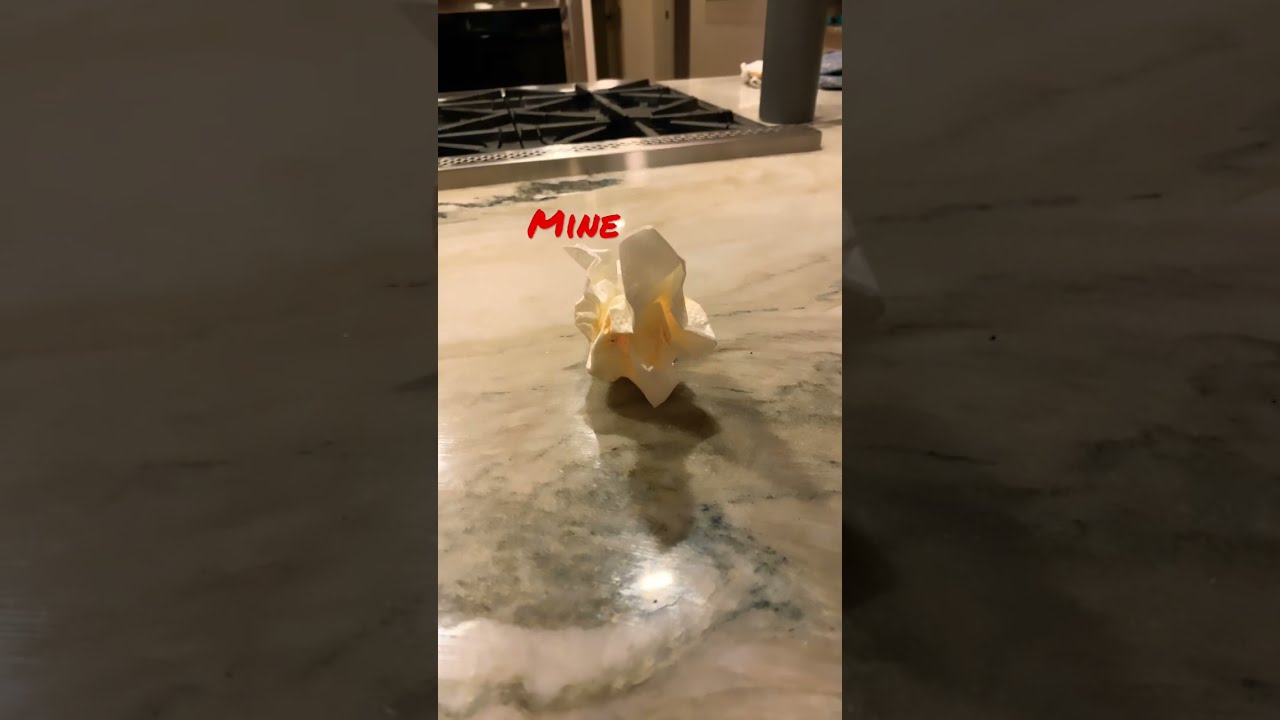The image captures a detailed view of a kitchen countertop, likely made of light-colored marble with dark gray veins. The center focus of the image appears to be a crumpled white paper napkin, giving off an origami-like appearance. Written across the napkin in bold red font is the word "MINE." The countertop reflects light from the kitchen, highlighting its polished surface. Behind the napkin, a gas stovetop with black grating and a silver bar is visible. Further in the background, there are glimpses of a cup, possibly some food on a plate, and a closed oven door against the far wall. The left and right edges of the image are dimmed, adding emphasis to the central countertop area. The photo seems to be a screenshot from a vertical video, likely from TikTok or Instagram Reels.